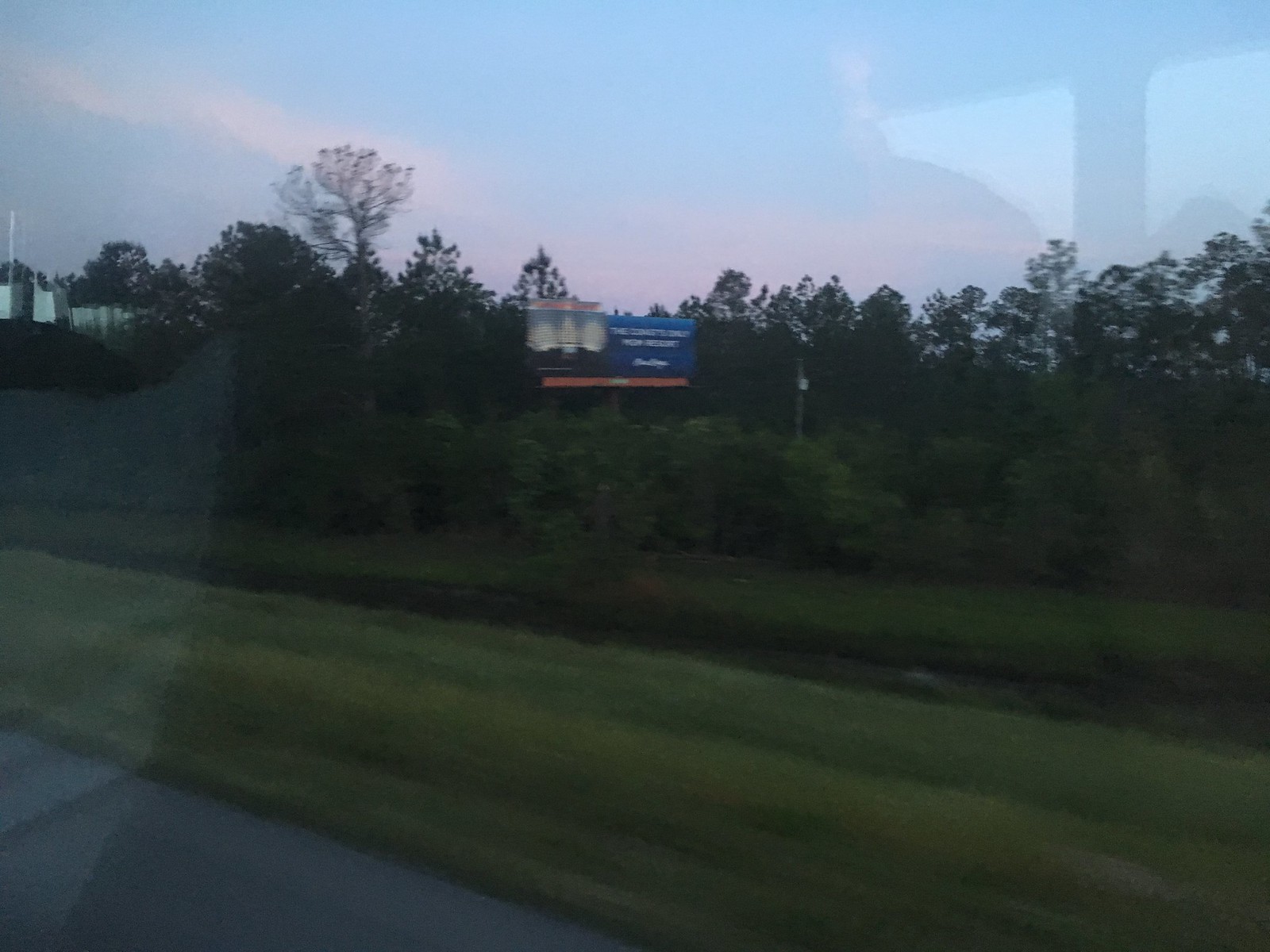The photograph captures a scene from inside a moving vehicle, potentially a bus, as inferred from the high vantage point. There is a noticeable reflection in the window, possibly of the vehicle's interior or an indistinct shape. The image features a roadside view characterized by a wide grassy strip followed by a stream or ditch, then another stretch of grass leading up to a thick tree line. Positioned in the tree line is a billboard that appears to be partially obscured and unreadable; the left side exhibits some form of image while the right side features a blue background with white text, and an orange border at the bottom. In the distance, at the far left corner of the photograph, small, white buildings are faintly visible against the backdrop of the woods. The upper segment of the image reveals a clear blue sky above the taller tree line. The overall image is imbued with reflections, adding a layer of complexity and obscuring some details.